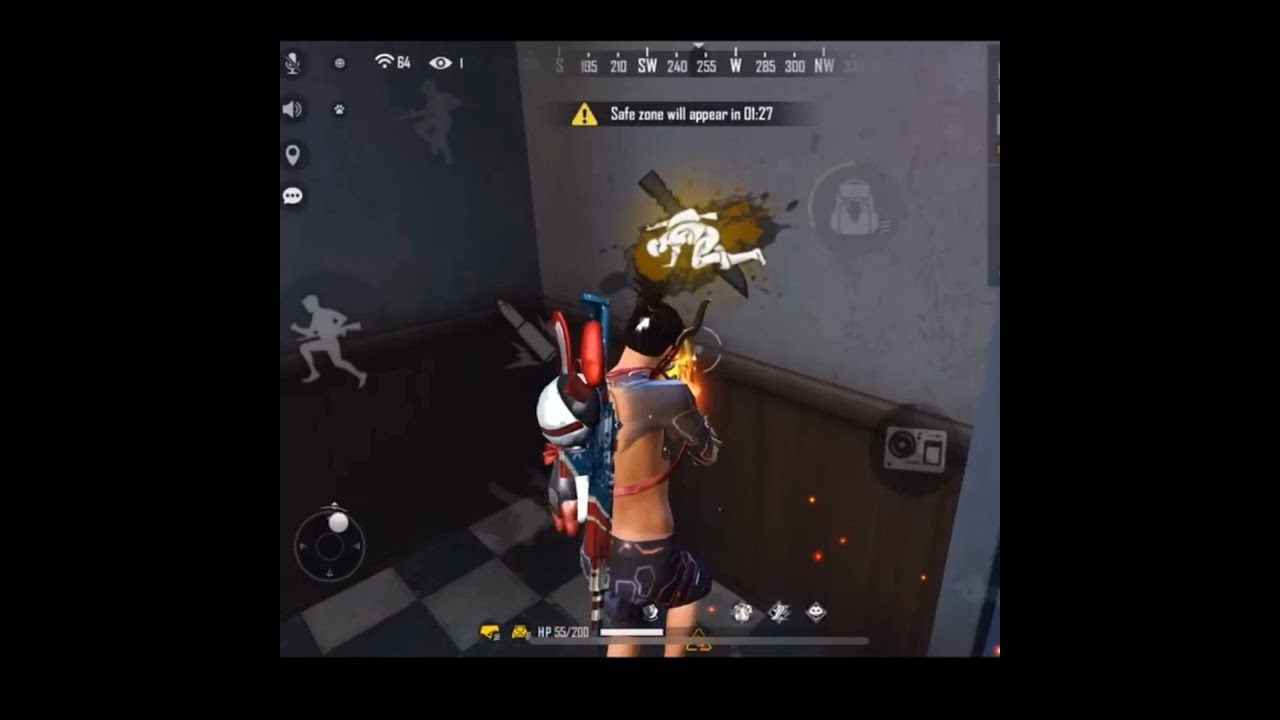This screenshot from a mobile third-person shooter video game captures an action-packed moment featuring a shirtless character equipped with an array of specialized gear. The avatar is donning black shorts and is adorned with shoulder armor and tattoos on his arms. Strapped to his back is a patriotic-themed arrangement of weaponry, including a helmet and gun, along with a red, black, and white bunny-shaped backpack. He is holding what appears to be a flamethrower or rifle. 

The game interface reveals a health meter showing 55 out of 200 points, and a compass at the top under which an alert indicates that a safe zone will appear in 1 minute and 27 seconds. The directional bar and several tabs for microphone, volume, map, and speaking surround the character. Additionally, a glowing icon on a nearby wall depicts a fallen soldier, emphasizing the game's focus on a dramatic, survivalist environment. This snapshot also highlights the network's connectivity through a Wi-Fi icon and features black panels on either side, indicative of the screen dimensions typically seen in mobile gaming.